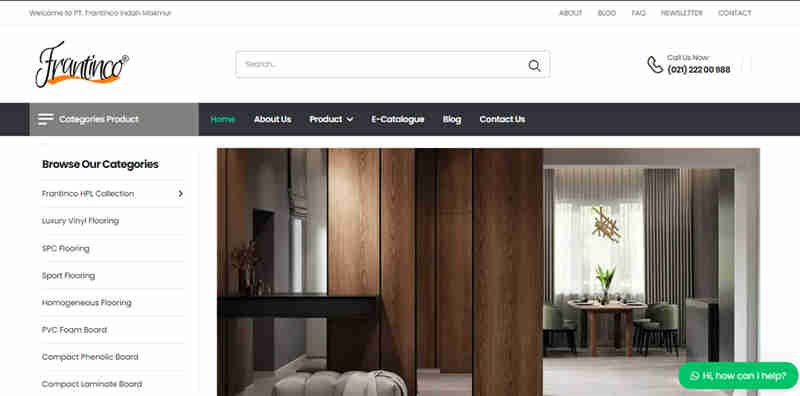This image is of a website with a rather blurry resolution, making the details difficult to discern. At the top, there's a thin black border running across the width of the page. The left side of the border contains the text "Welcome to" followed by an illegible, blurry section. On the right side of the border, in black lettering, there are clickable dropdown menu items that read "About," "FAQ," "Newsletter," and "Contact."

Beneath the "Newsletter" option, the text "Call Us Now" is displayed, accompanied by a bolded phone number. To the left of this phone number is a phone icon with a black border and a white interior. Further left, there's a large search bar. On the left corner of the page, the website name "Frantico" is present, underlined with a wavy green line.

Below this, there is a half-inch tall black border followed by a gray section that begins about half an inch in. This gray section contains categories labeled "Categories," "Product," and, in green, "Home." Additional menu items in white include "About Us," "Product," "e-Catalog," "Blog," and "Contact Us."

Underneath the "Home" menu item, an image of a room is displayed. The room features wood-paneled walls on the left side with a window, a table, and a green carpet on the right side. In the bottom left corner of this image, there is a green tab with white text that reads, "Hi, how can I help you?"

Below the gray section, the lower part of the page is white, with a bolded black heading that says "Browse Our Categories" located about two inches from the left margin. There are eight clickable options available for browsing different categories.